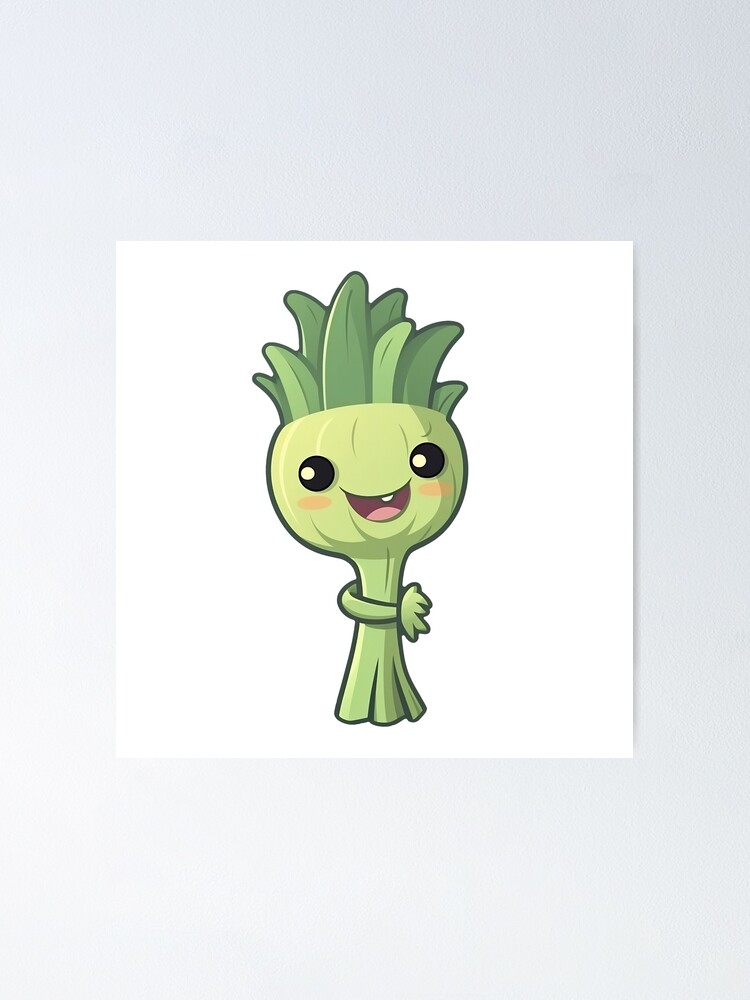This detailed digital illustration features a cute animated character resembling a baby leek or plant. The character is primarily green, with various shades adding depth. Its body is thin, akin to a stem, with a cutout at the bottom to represent legs and is flanked by what look like small hand-like branches serving as arms. This whimsical figure is set against a white square poster background that contrasts with a subtle grey surface behind it. 

Its head is bulbous, forming the top of the leek, adorned with green leaf-like hair. The face is expressive, featuring large black eyes with smaller white circles, giving it a vivid and endearing appearance. Below the eyes, there are orange blush spots adding a touch of warmth. The open mouth shows a single tooth in the center, complemented by a visible pink tongue, suggesting a cheerful, friendly demeanor. The overall design of the character is aimed at invoking the charm and happiness of a baby vegetable, likely intended for a cartoon or animated series.